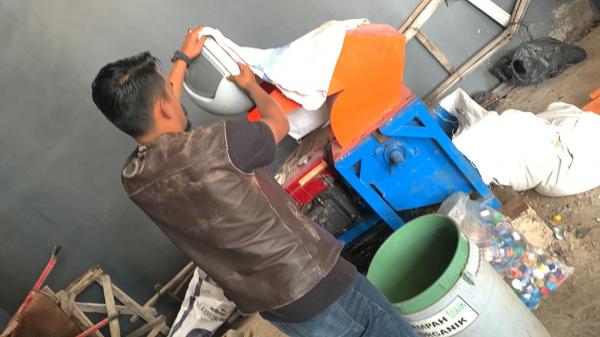In this image, a man with dark tan skin and black hair is depicted working in a factory-like setting with a dirt floor. He is dressed in a brown leather vest over a grey t-shirt and blue jeans, complemented by a black wristwatch on his left wrist. The man stands at a steel table that features a blue section with a red countertop, where an orange arm extends, serving as a support for the item he is working on.

The item appears to be a trash lid with a small movable panel, which the man is polishing with a rug. The orange arm of the table holds the trash lid in place as he cleans. In front of him, there is a green pail and another grey bucket, with some black trash bags and sacks scattered on the ground. Additionally, a plastic bag containing red, white, black, and orange pieces is situated in front of the pail. Leaned against the grey wall in front of him is a steel ladder, and to the side, a wooden ladder also rests against the wall. The scene captures the industrious atmosphere typical of such a work environment.